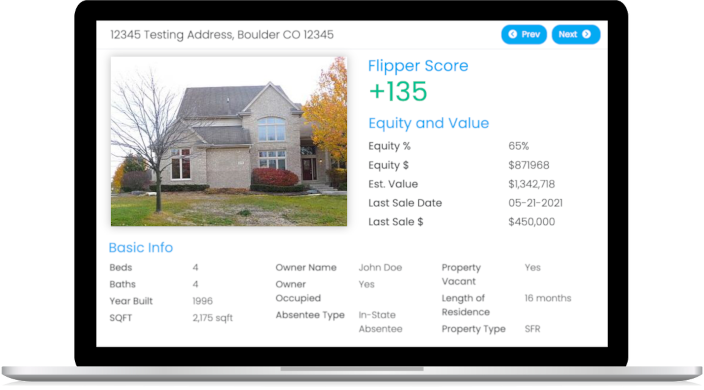The image showcases a laptop screen displaying detailed real estate information. Central to the screen is a file directory named "Testing Address Folder Colorado CO," which includes five entries labeled from 1 to 5. 

At the top are navigation controls with a blue oval containing a "PREV" button accompanied by a left arrow, and a "NEXT" button coupled with a right arrow—both text elements are in white. 

Adjacent to the address folder is a photograph of a two-story brick house. 

The screen also highlights several metrics, including a "Flipper Score" of +135 in green, the value breakdown of which appears in blue text. "Equity" is divided into two sections: one showing a percentage of "65%" and the other a monetary value of "$871,968." The "Estimated Value" is noted as "$1,342,718."

Furthermore, the display records the "Last Sale Date" as May 21, 2021, with a "Last Sale Price" of $450,000. Essential property details in blue text include "Beds: 4," "Baths: 4," "Year Built: 1996," and "Square Feet: 2,175 sqft."